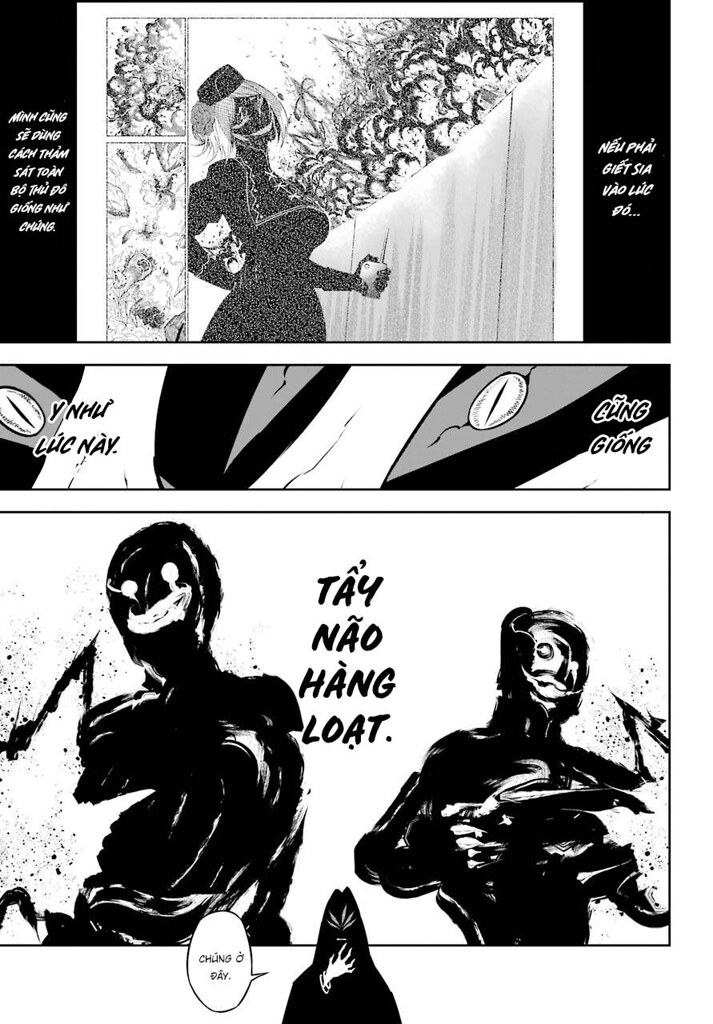This black and white image, presented in the style of comic book art, features three distinct frames with Vietnamese text accompanying the visuals. In the top frame, a woman dressed entirely in black holds a remote, potentially detonating an explosion. Her face is obscured, with only her white eyes and mouth visible, creating a dramatic contrast. The middle frame is more abstract, possibly depicting just a pair of eyes set against a dark background. The bottom frame shows two figures, both in all-black attire with simplistic white faces, their eyes and smiles starkly drawn. Additionally, these figures appear to be shooting firearms. Together, these frames create a gripping, suspenseful narrative that is deeply embedded in comic traditions and enhanced by the enigmatic use of black and white.